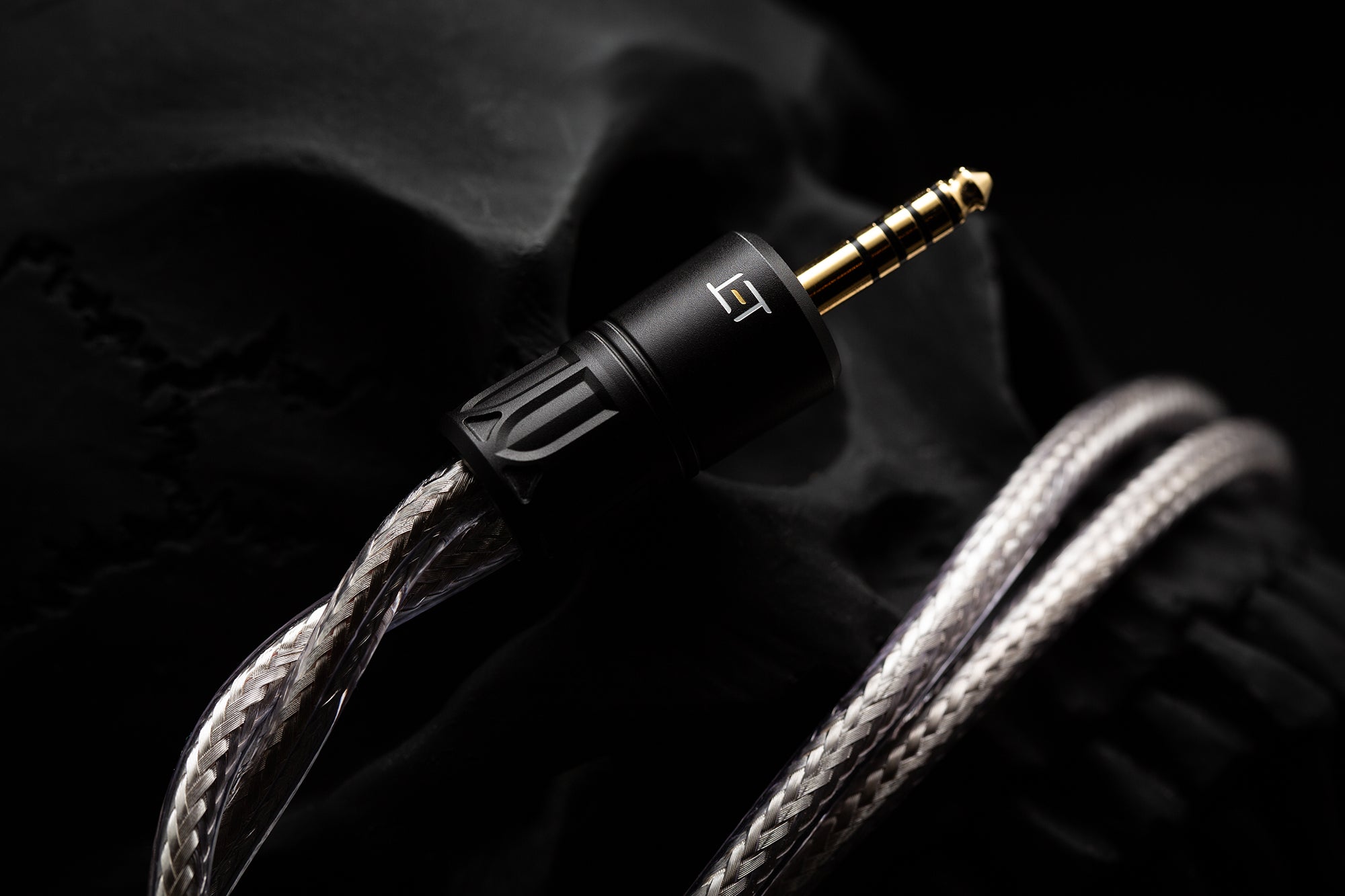This image is a professionally taken, close-up photograph reminiscent of a catalog or product advertisement, centered around a 3.5mm auxiliary audio connector. The standout element is the metallic, braided cord wrapped in clear plastic. The audio connector, likely used for studio equipment or headphones, terminates in a black plastic knob. This knob features an emblem composed of two straight, mirrored lines with a yellow dash in the middle, forming the letters 'L' and 'T' or a square symbol. The image is set against a completely black background, enhancing the dramatic effect created by the dark, 3D-printed black plastic skull in the frame. The skull, faded and distant, with large open eye sockets and visible cracks on the left side, adds an intriguing and edgy juxtaposition. Light from the left side of the photo highlights the skull's intricate details. The cable strategically wraps twice around the skull, positioned below the nose and above the teeth, leading to the brass-colored insertion point marked with brown strips that denote the correct depth for connection.